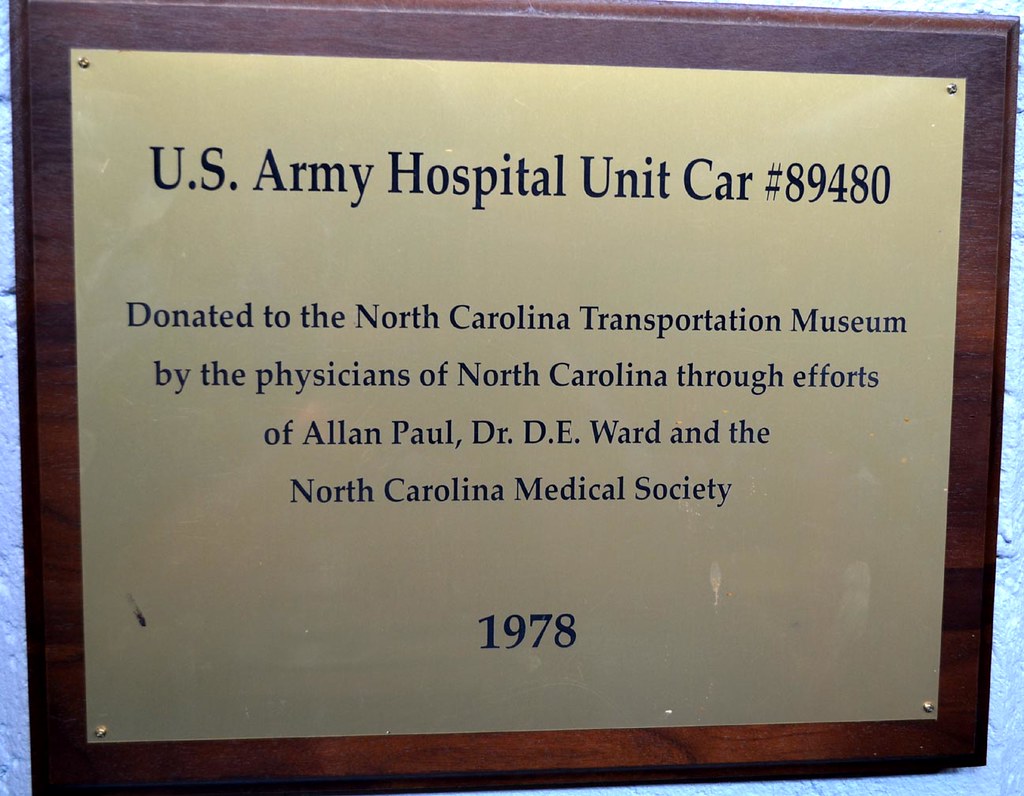Mounted on a cinder block wall, there is an attractive wooden placard with a dark stain, encased in a slightly rectangular wooden frame. Fixed to this frame with bolts at each corner is a gold-toned metal plaque with embossed dark blue lettering. The plaque reads: "U.S. Army Hospital Unit Car number 89480." After a small space, the text continues: "Donated to the North Carolina Transportation Museum by the Physicians of North Carolina through efforts of Alan Paul, Dr. D.E. Ward, and the North Carolina Medical Society." At the very bottom, there is the year "1978," possibly in a slightly larger or darker font. Despite a few minor scratches, the placard remains in good condition and is quite visually appealing.